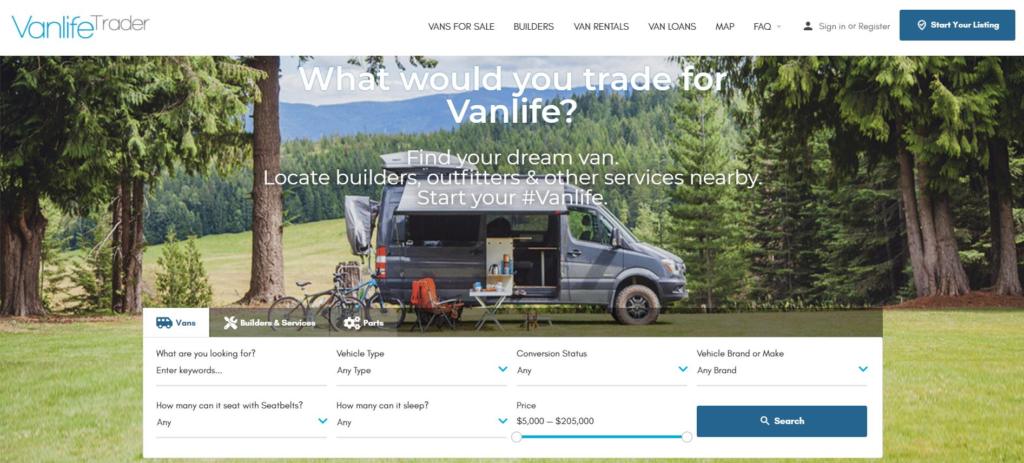This detailed caption summarizes the various elements present on a webpage from VanLifeTrader.com, highlighting its structure and key features:

---

This image captures the top section of the Van Life Trader website, an online platform dedicated to the van life community. The header of the site features tabs for various sections: **Vans for Sale**, **Builders**, **Van Rentals**, **Van Loaning**, **Van Loans**, **Map**, and **FAQ**, accompanied by a user icon with options to sign in or register.

Beneath the main navigation is a prominent blue tab with a check icon, labeled "Start Your Journey." Central to the image is a scenic photograph of a campsite, situated in a wooded area away from any urban landscape, surrounded by lush trees and grass. A gray van with lighter gray accents is parked at the site, showcasing an open door, an awning providing shade, a set of outdoor table and chairs, a couple of bicycles, and a functional luggage rack on top.

Overlaying this picturesque scene is the text: "What Would You Trade For Van Life? Find your dream van, locate builders, outfitters, and other services nearby. Start your hashtag #VanLife."

Below this, a search box invites users to find vans, prompting them to select specifications such as conversion status, brand, make, and keywords. Dropdown menus allow selection by seating capacity with seatbelts, sleeping capacity, and price range listed from $5,000 to $205,000, followed by a prominent "Search" button.

--- 

This detailed description provides a comprehensive insight into the visual layout and functionality of the top section of the Van Life Trader website.